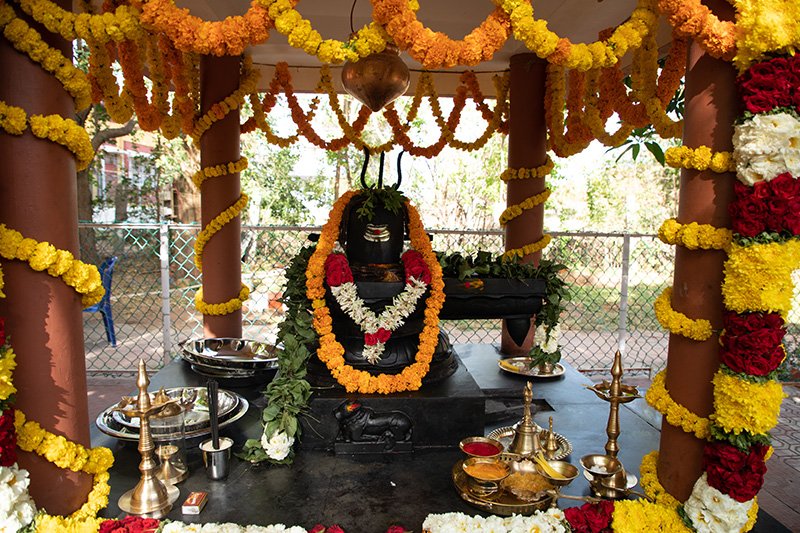This image captures a vibrant, outdoor ceremonial shrine, potentially situated in East Asia, Thailand, India, or Bali. The shrine is sheltered within a gazebo-like pavilion, supported by four ornamented pillars. Each pillar is abundantly wrapped in garlands of colorful flowers, predominantly in yellow, orange, white, and red hues. Additional flowers drape in decorative loops from the pavilion’s roof. 

At the heart of the shrine, a black stone statue of a seated figure commands attention, adorned with multiple garlands of orange, red, and white flowers around its neck and head. Surrounding the base of the statue is an assortment of ceremonial items, including metal trays that hold bowls of what appears to be food offerings, incense burners, ornate metal dishes, spices, and a bell. A box of matches is also visible in the forefront.

In the backdrop, a chain link fence is seen, along with a building and several trees, enriching the natural and tranquil ambiance. The variety of elements suggests a celebration or festivity, likely a significant traditional or religious event to honor an important figure.